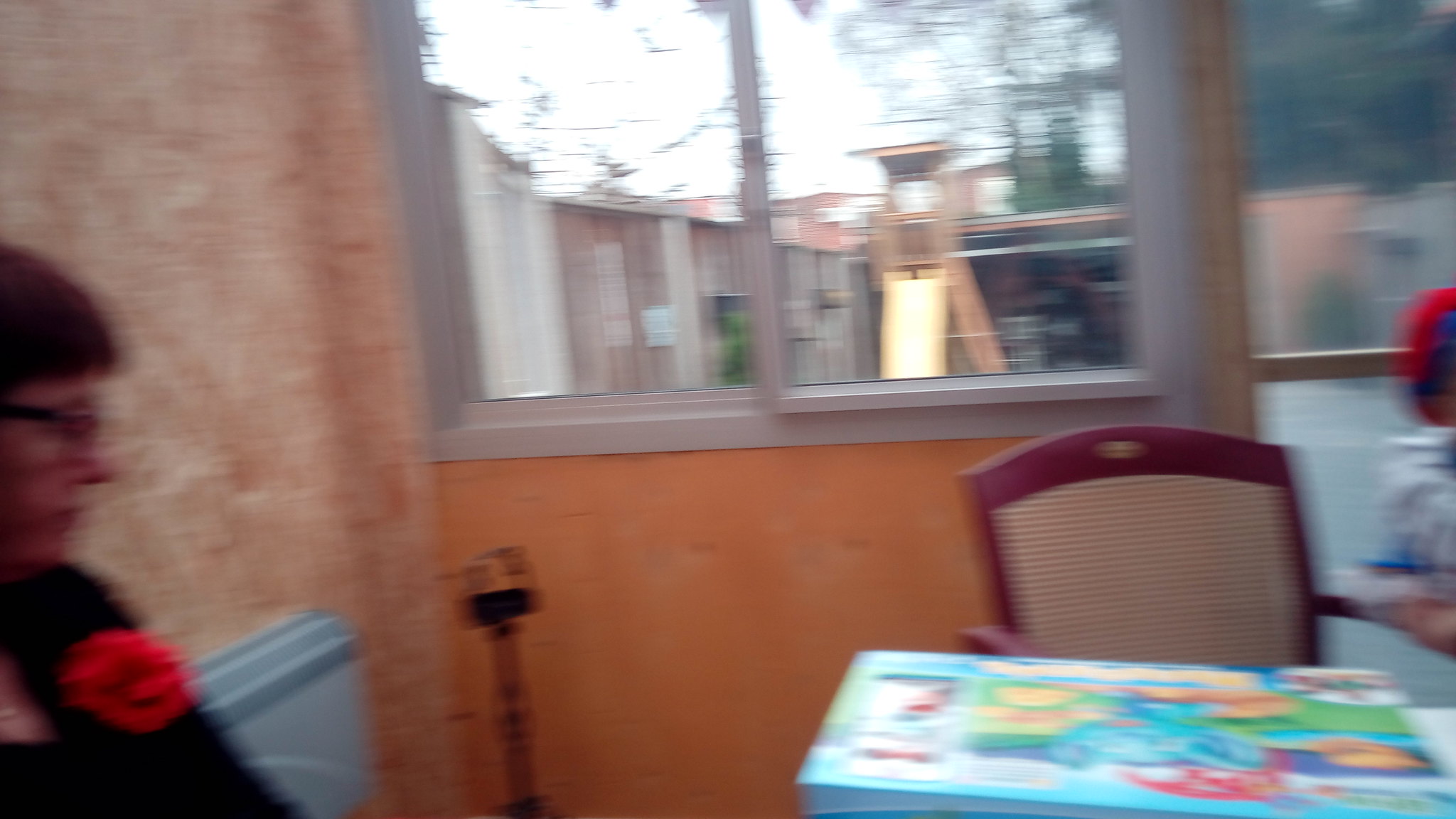This photograph captures the interior of a waiting room or restaurant, characterized by its wooden architecture. To the left, a lady sits on an attached blue bench. She is adorned in a black jacket featuring a striking red flower corsage on the front, and she wears black glasses. Her gaze is directed towards the right side of the frame. Adjacent to her, there is a table topped with a large, square blue box. Behind the table stands a burgundy-colored chair, distinctive with its wooden arms and cloth upholstery in the middle of the backrest. The background reveals two windows, one of which slides back behind the other, further emphasizing the wooden structure of the building.